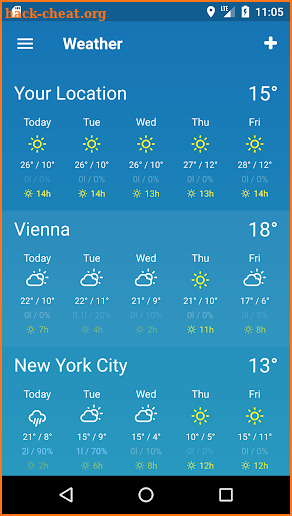The image is a detailed screenshot of a weather app displayed on someone's phone. At the top of the screen, a dark blue menu bar features several icons: a page icon on the left and a series of status indicators on the right, including a map pinpoint logo, an LTE signal indicator, a battery bar with a lightning bolt, and the current time, which is 11:05. The screenshot is highlighted by an orange border with a watermark reading "hack-cheat.org" in the top-left corner, directly above the page icon.

Below the menu bar, the weather app interface begins with a trio of horizontal lines on the top left to signify a menu, followed by the word "Weather" in bold white font in the center. To the right, there is a white plus sign. The main content of the app is divided into three sections. 

The first section, labeled "Your Location," shows a current temperature of 15 degrees and provides a five-day forecast. Each day is represented by an icon depicting the predicted weather conditions, with details on daily highs, lows, and sunshine duration.

The second section, with a slightly different blue hue, is labeled "Vienna." It displays a current temperature of 18 degrees and includes a five-day forecast. Unlike "Your Location," this section shows a mix of sun and clouds.

The third section is dedicated to "New York City," where the current temperature is noted as 13 degrees. The five-day forecast here shows a varied weather pattern, starting with rain and clouds on the first day and transitioning to partly cloudy skies and sunshine on subsequent days.

At the bottom of the page, the phone’s navigation bar includes three icons: a left-pointing arrow for back navigation, a circle for the home screen, and a square for recent apps.